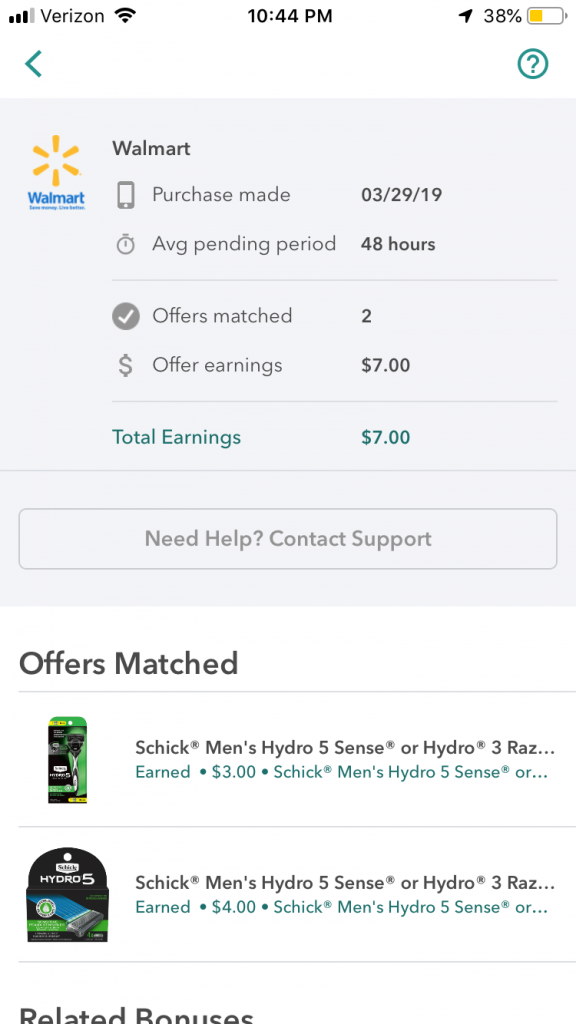In this screenshot of a mobile device, the top left corner displays the network signal bar at three out of four strength points, indicating a fairly strong connection. Next to the signal strength, the network provider "Verizon" is mentioned. Adjacent to this, the Wi-Fi signal is fully engaged, showing three out of three bars, denoting an excellent wireless connection. 

Moving towards the center-top, the current time is displayed, reading 10:44 PM. On the top right, several icons are visible: a location icon, which signifies that location services are active, and a battery icon showing a 38% charge remaining.

Below these status indicators, there is text pertaining to a recent transaction: it reads "Walmart," denoting the retailer. The purchase date is listed as 03-29-2019, followed by the note "average pending period 48 hours," implying a standard processing time. The specific matched offer is detailed as providing earnings of $7, which also represents the total earnings shown.